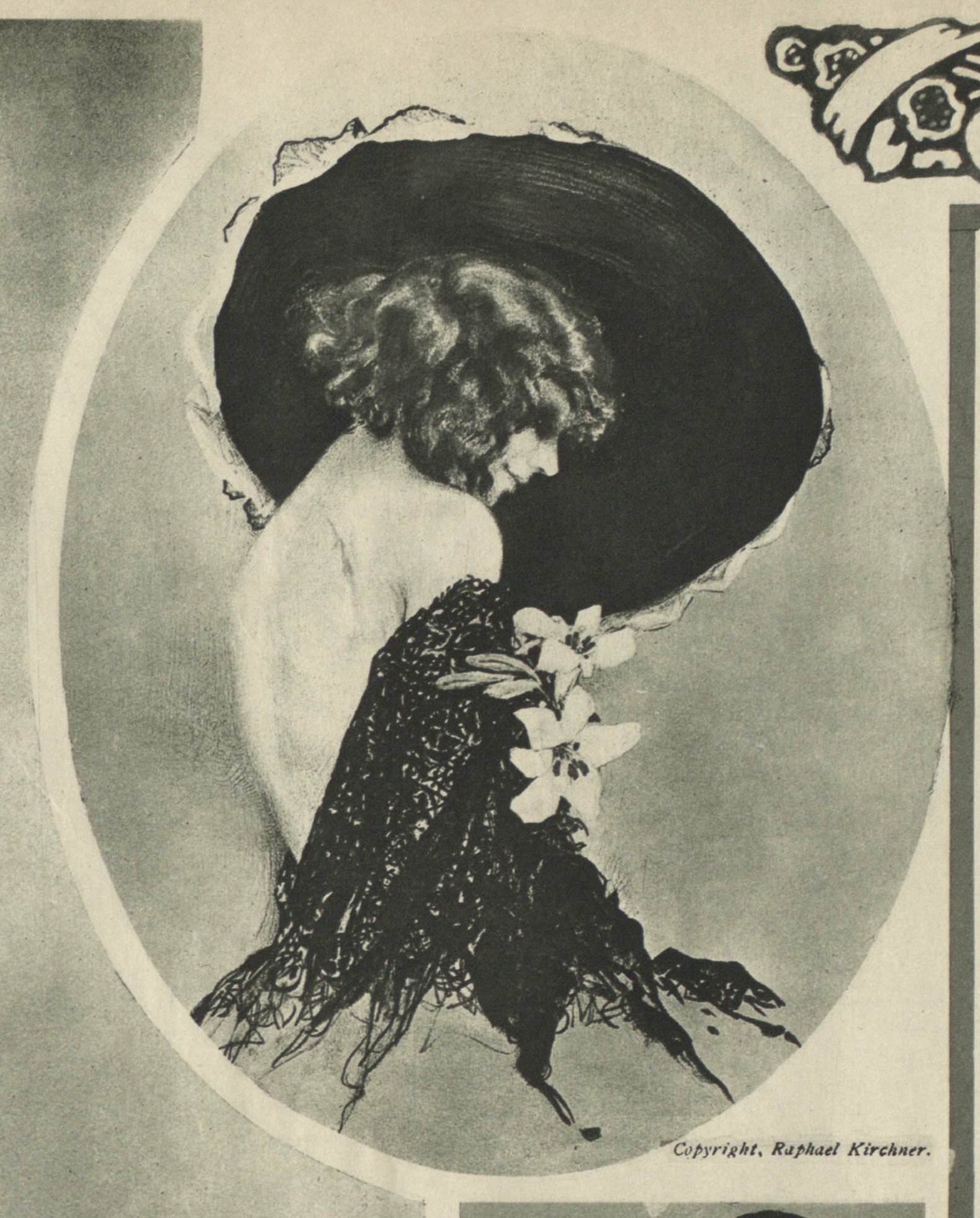The image is a black and white illustration by Raphael Kirchner, with copyright indicated at the bottom. The artwork, likely from the 1910s to 1930s, features a stylish lady seated in a side pose within an oval frame. Her right shoulder and back are exposed, as she wears only a black shawl with fringes draped over her right arm. She has short, curly hair that appears either black or brown and a slight, intimate smile on her face. The woman holds two large white lilies with black centers near her elbow. Atop her head, a large black hat with lace or ruffle trim is tipped back, revealing just a bit of its decorative edge. The entire image is rendered in varying shades of gray, capturing a vintage charm and possibly suggesting its use for illustration or advertising purposes. The composite framing includes some form of design in the top right corner, adding to its aesthetic appeal.